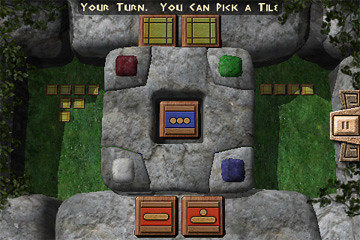The image appears to depict a computer game interface. At the top of the screen, the text "Your Turn" is prominently displayed, indicating that it is the player's move. The top edge of the screen is adorned with a row of rocks, framing the display. Central to the image is a large, rock-like square. Each corner of this square contains a different colored button, each shaded uniquely: a red square in the top left, a green square in the top right, a white square in the bottom left, and a purple square in the bottom right. In the middle of the main square, there is another square that features three round shapes.

The bottom of the screen is also lined with rocks, and contains several selectable red boxes, likely representing different options or actions the player can take. The right side of the screen is bordered with rocks as well, incorporating a play/pause button for game control. Surrounding this rocky interface are patches of turf interspersed with small tiles, adding texture to the overall design.